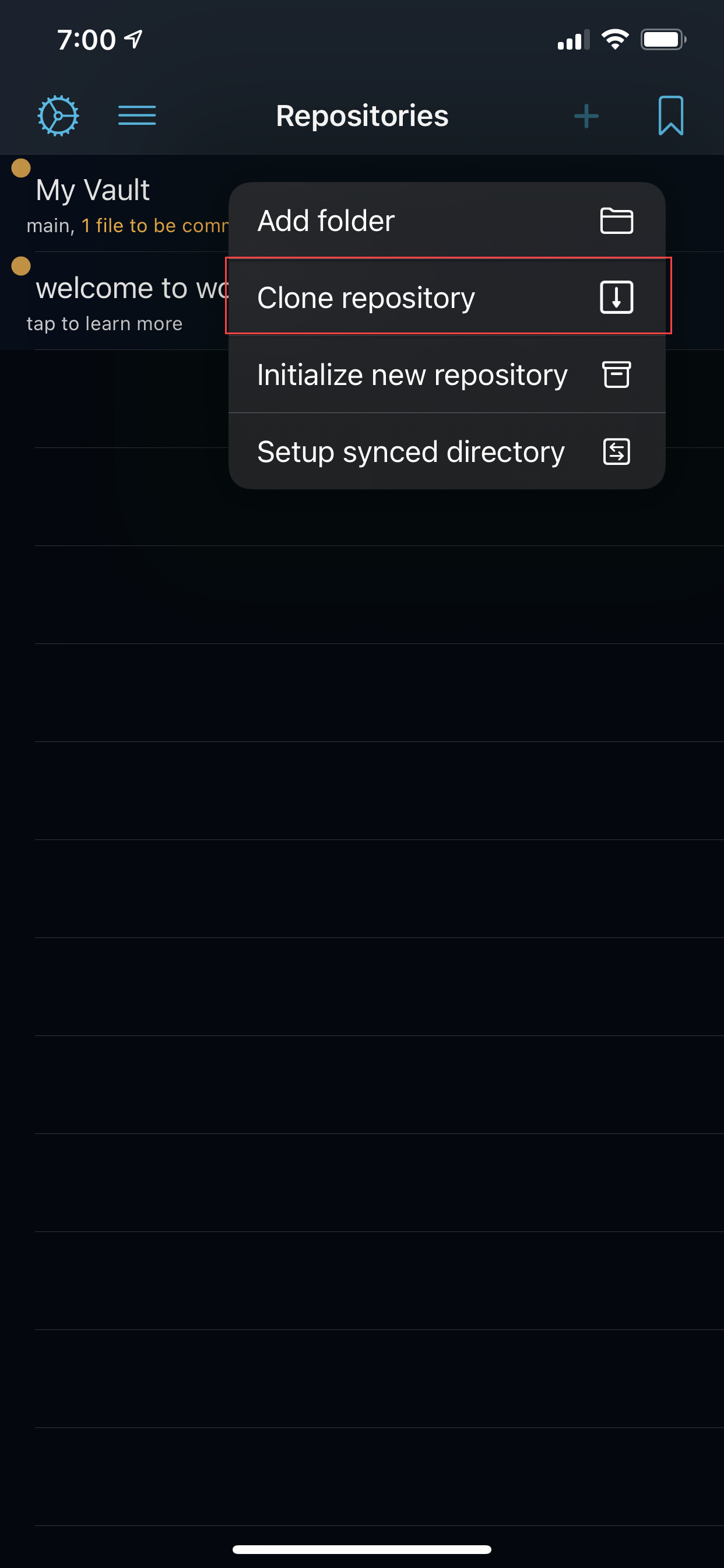The screenshot captures the interface of a cell phone at 7 p.m., as indicated by the time display at the top. Adjacent to the time, there is a navigation symbol, showing the phone's active navigation mode. The status bar also reveals that the phone has three bars of signal strength, is connected to Wi-Fi, and possesses a fully charged battery. The device is set in dark mode, providing a sleek, nighttime-friendly display.

The user is interacting within an application related to file management or settings, as suggested by the visible options beneath the status bar. Dominating the screen is a drop-down menu within a section labeled "Repositories." The options available in this menu include "Add Folder," "Clone Repository," "Initialize New Repository," and "Set Up Sync Directory." At this moment, the user has highlighted or selected "Clone Repository."

Behind this menu, partially visible text indicates two items: one labeled "My vault main one file to be..." and another that starts with "Welcome to WO..." Both entries are accompanied by dot indicators, suggesting unread notifications or updates pertaining to the app. Additionally, the "Welcome to WO..." text includes a clickable instruction to "Tap to learn more."